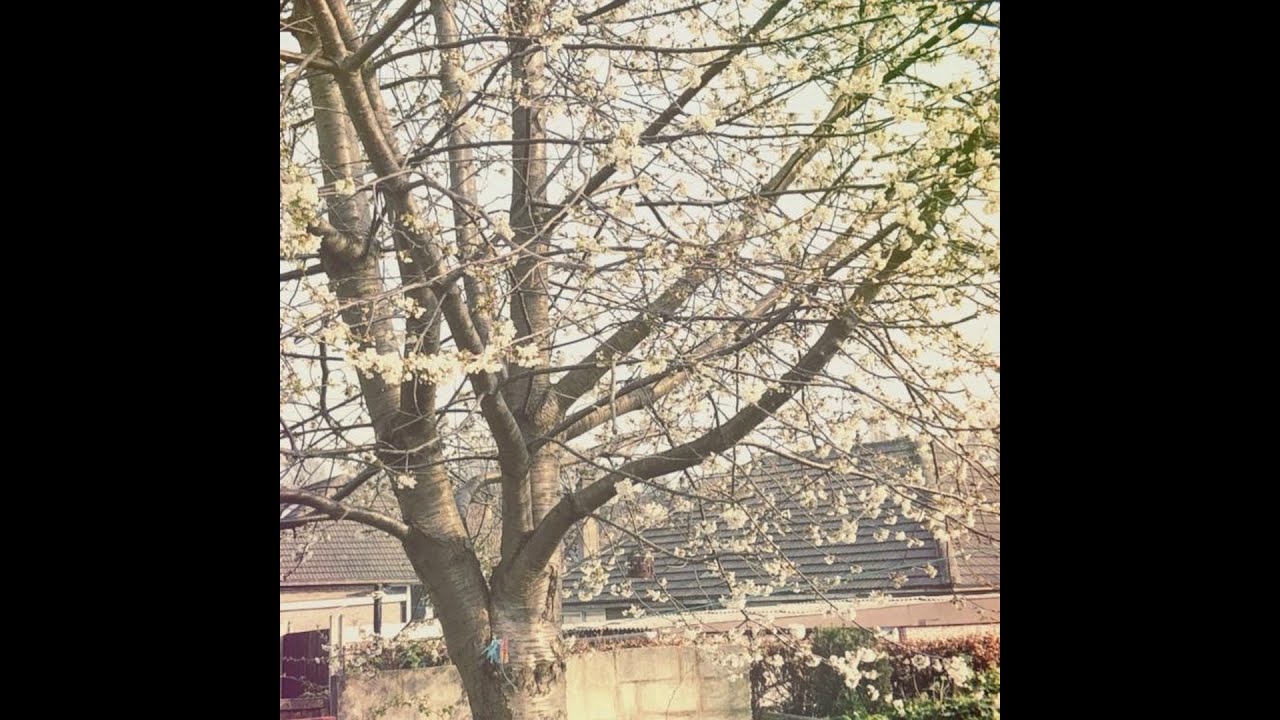The image portrays a tree, slightly left of center, extending vertically from the bottom to the top of the frame. The slender, spindly branches are adorned with numerous small, white flowers, suggesting the tree could be a dogwood in full bloom, indicative of springtime. The tree is set against a light gray, overcast sky, contributing to a subdued atmosphere. Behind the tree, two houses with gray roofs form the backdrop, accompanied by a whitish-gray cement wall at the lower part of the frame, likely separating backyards in the neighborhood. The yellowed tint of the photo gives it a slightly aged appearance, adding to its charm. Some additional plants and flowers are visible at the lower right corner, completing the scene.